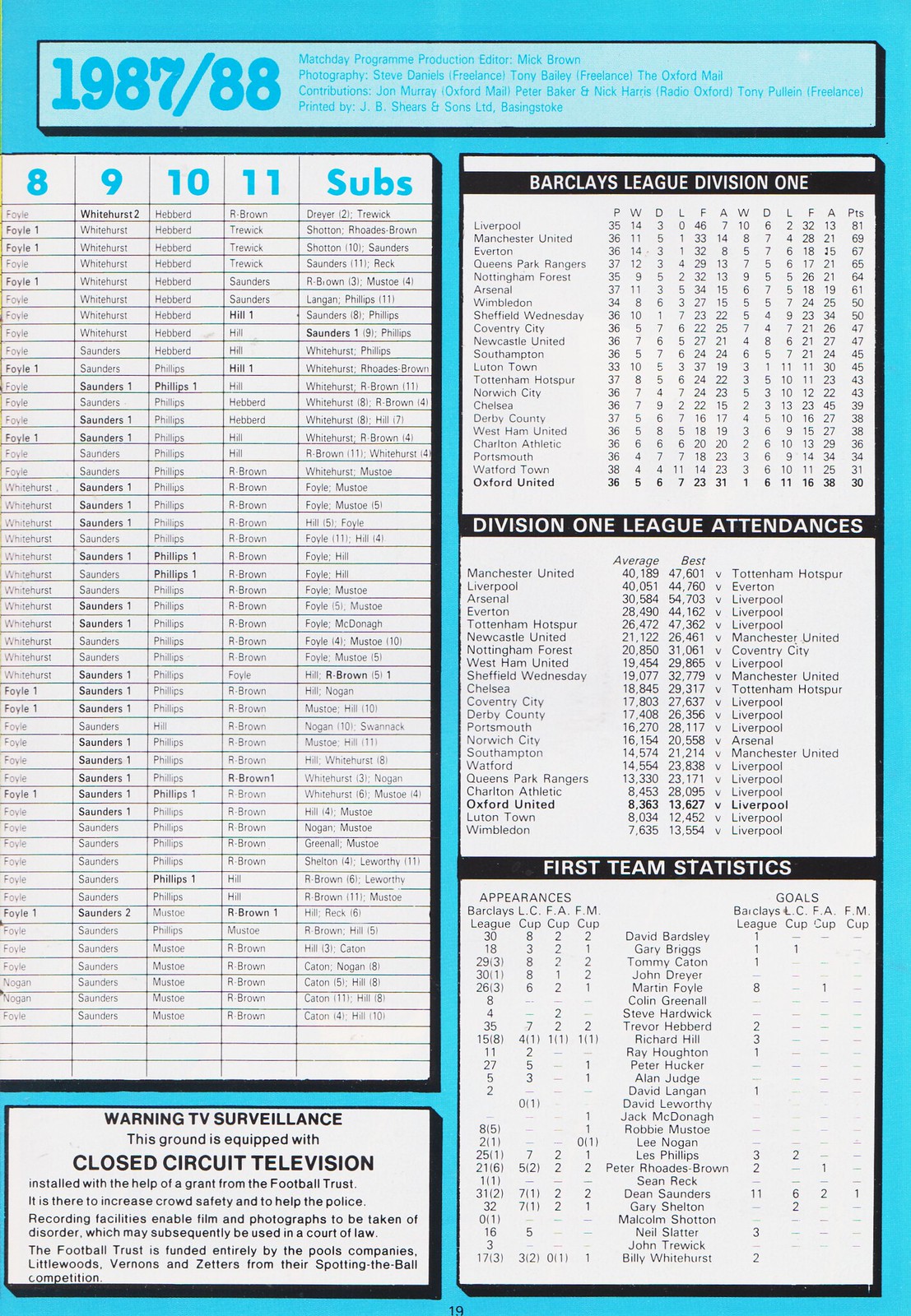The image displays a single sheet of paper, seemingly a page from an old game day program, likely from the 1987-88 Barclays League Division 1 season. The page is filled with text and tables against a black, white, and light blue color scheme. At the top, it credits Mick Brown as the Match Day Program Production Editor and Steve Daniels for photography. The content includes various contributors and significant football statistics and details. 

On the left side of the page, there's a partial table starting with columns numbered 8, 9, 10, 11, and a "subs" column, filled with player names. At the bottom left, a notice reads: "Warning, TV Surveillance. This ground is equipped with closed circuit television, installed with the help of a grant from Football Trust." 

The right side of the page features three distinct tables: The first titled "Barclays League Division 1" lists teams along with their respective statistics. The second table, labeled "Division 1 League Attendances," displays average and best attendance figures per team. The final table, "First Team Statistics," provides a comprehensive list of stats related to first-team players and performances. The overall style suggests this was part of a pre-game program outlining important game details and team information.